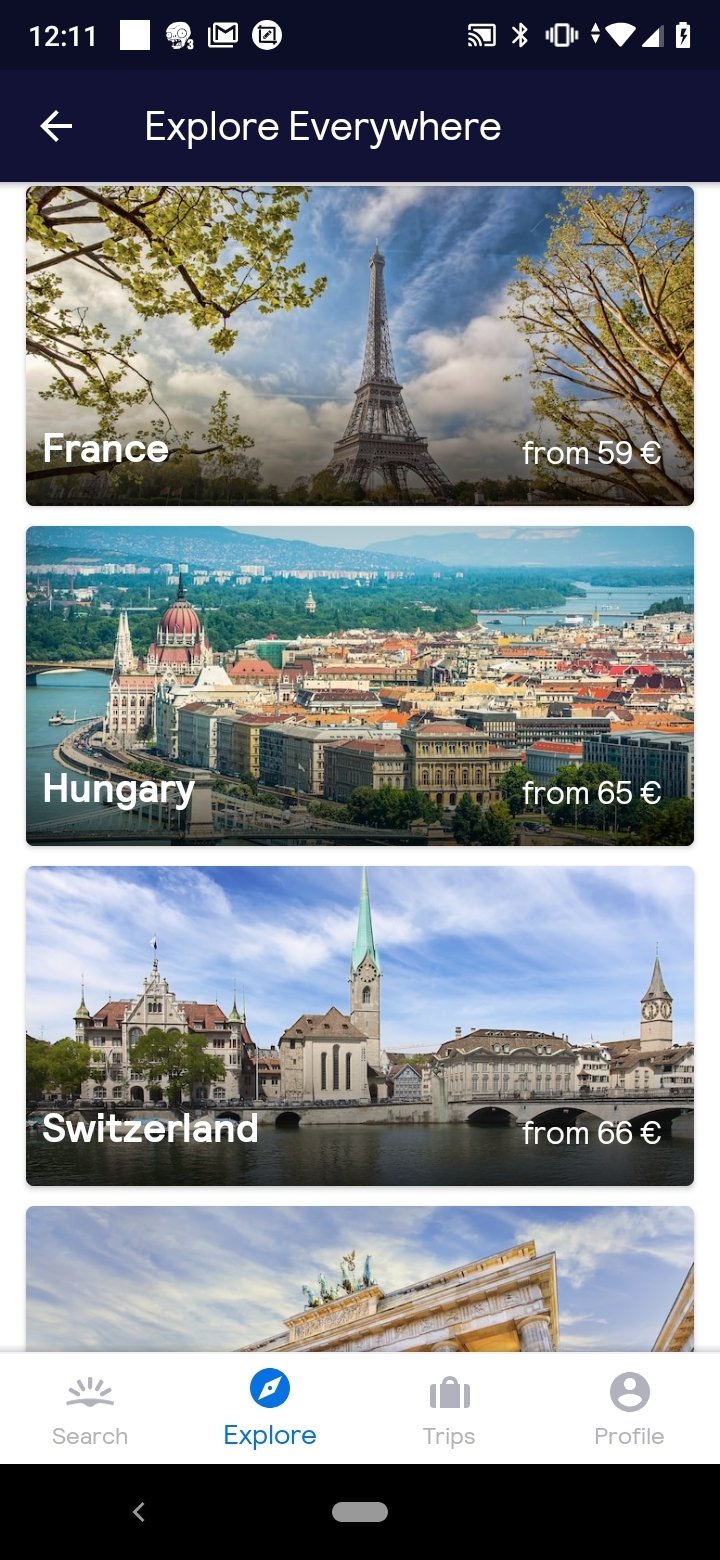The image features a travel-themed interface with various elements displayed prominently. At the top, there is a Bluetooth symbol next to battery indicators showing a charge level. A blue bar with the phrase "Explore Everywhere" and an arrow pointing to the left is also visible.

In the center of the image, there are several photographs of famous landmarks and cities, each accompanied by a price tag in euros. One image displays the Eiffel Tower in France, marked at 59 Euros. Another shows a cityscape labeled "Hungary," priced at 65 Euros, and a different image features numerous buildings in Switzerland, also for 65 Euros. 

An additional picture is divided horizontally, displaying the top of a building and a search bar underneath. To the right of this, there is an icon of a sun and the word "Explore" in blue, accompanied by a compass icon.

At the bottom portion of the interface, navigation icons including "Trips" (depicted with a suitcase), "Profile" (shown with a blank profile picture), and other unspecified icons are listed. The very bottom of the image is black, containing a left-facing arrow and a gray bar.